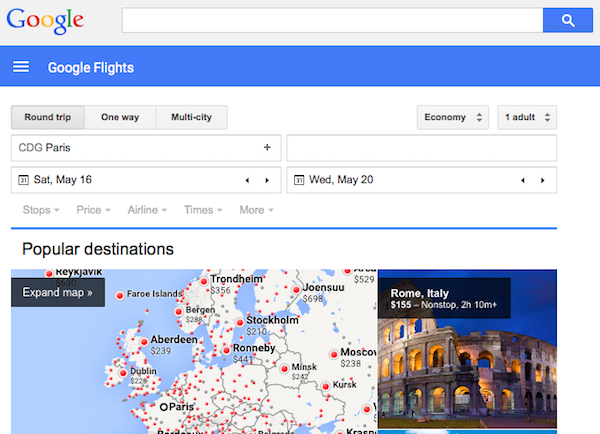This is a detailed screenshot of Google Maps integrated with Google Flights. At the top of the page, the iconic Google logo is prominently displayed, featuring its distinctive blue, red, yellow, green, and red colors. Below the logo is a search bar with a magnifying glass icon on the left side. Immediately underneath, there is a blue navigation bar with three horizontal lines on the right, followed by the text "Google Flights."

The main content shows a search interface for flights. A user has initiated a search for flights departing from Paris, as indicated by the first search bar labeled "CDG Paris." The destination search bar is currently blank, suggesting the user has not yet specified the destination. Below the search bars, the specified trip details indicate a round-trip, economy class for one adult, with departure on Saturday, May 16th, and return on Wednesday, May 20th.

Further down, there are filter options for stops, price, airline, times, and more, all of which are grayed out, indicating they are available for selection. 

The section labeled "Popular Destinations" showcases a detailed map of Europe with numerous red dots indicating possible destinations accessible from Paris. Notable destination markers include Reykjavik, Aberdeen, Dublin, Stockholm, Trondheim, Moscow, Kursk, and Minsk. Each red dot represents a different potential airport.

On the left side of this map, there is a highlighted destination offering: a flight to Rome, Italy, priced at $155 for a non-stop journey lasting two hours and ten minutes. An illustrative image accompanies this suggestion, depicting the ancient ruins of the Colosseum against a backdrop of blue sky, with the structure lit warmly from the inside.

Overall, the screenshot presents a comprehensive view of the flight search process on Google Flights, with visual and textual elements clearly guiding the user through the interface.